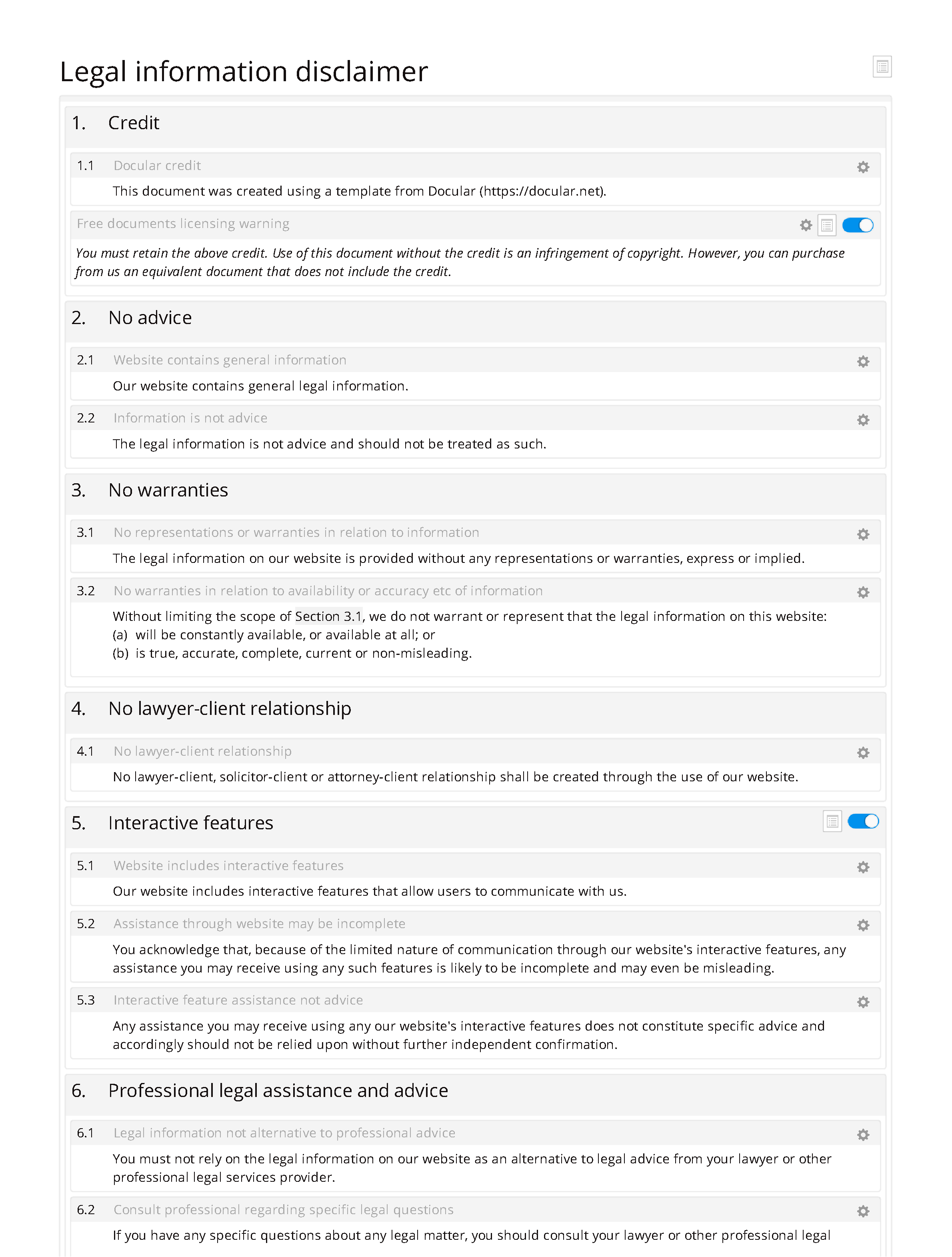The image features a blue and white background with a header that reads "Legal Information Disclaimer." Below the header, the content is organized into numbered sections highlighted in blue boxes. 

1. **Credit** 
   - A blue box labeled "1" contains the word "Credit."
   - Adjacent to it, there is a white box with informational text.
   - Included in this section is a small circle and a blue toggle switch.

2. **No Advice**
   - A blue box labeled "2" contains the phrase "No Advice."
   - It features a white box with a line and a small circle at the end.
   - The subsequent line also has a small circle.

3. **No Warranties**
   - A blue box labeled "3" contains the phrase "No Warranties."
   - Includes sub-sections 2.1 and 3.2, each with lines, small dots, and circles.

4. **No Lawyer-Client Relationship**
   - A blue box labeled "4" contains the phrase "No Lawyer-Client Relationship."
   - This section consists of multiple lines with small circles interspersed, illustrating different points.

5. **Interactive Features**
   - A blue box labeled "5" highlights "Interactive Features."
   - This section includes a blue toggle switch.
   - Additionally, there are three lines, each terminating in small circles.

6. **Professional Legal Assistance and Advice**
   - A blue box labeled "6" contains the phrase "Professional Legal Assistance and Advice."
   - This final section includes two lines, each ending in small circles on the right.

Overall, the image provides a detailed disclaimer with distinct sections, each clearly marked and illustrated with lines, circles, dots, and toggle switches for emphasis.